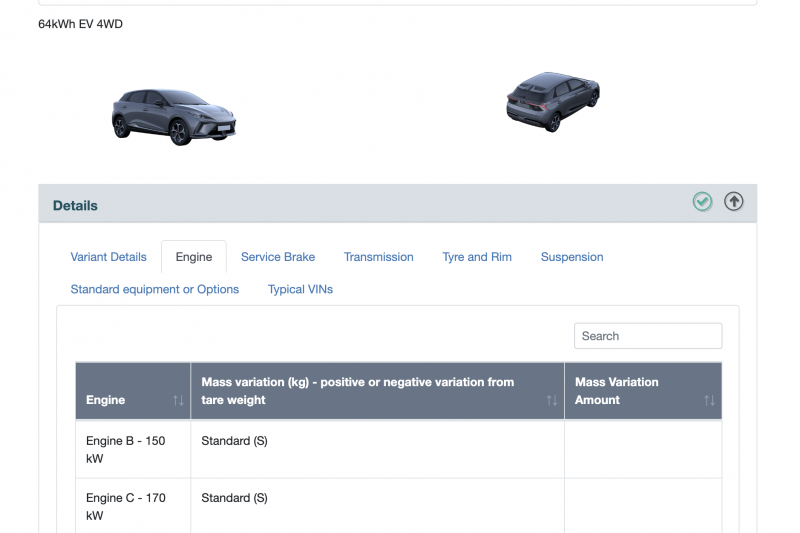This is a screenshot of a website interface. The background is primarily white, particularly noticeable in the upper left corner where the text "64KWHEV for WD" is displayed. Directly below this, there are two small graphics depicting a blue hatchback SUV against a white background.

Below these graphics, a gray bar appears on the left side with the word "Details" prominently shown in black font. To the right of the gray bar, there are two circles: one containing a check mark and the other featuring an upward-pointing arrow.

Beneath this section, a white background hosts text in blue font that reads "Variant Details Engine." This section is currently selected, indicated by its black coloration. Adjacent to this section are other menu options: Service Brakes, Transmissions, Tire and Rim, Suspension, Standard Equipment, Options, and Typical VINS.

A table is presented below these options. At the top of the table, a gray rectangle lists the column headings: "Engine," "Mass Variation (kg)," "Positive or Negative Variation from Tare Weight," and to the right, "Mass Variation Amount." Underneath the "Engine" column, the entries are as follows: "Engine B, 150 kW, Standard S" and "Engine C, 170 kW, Standard S."